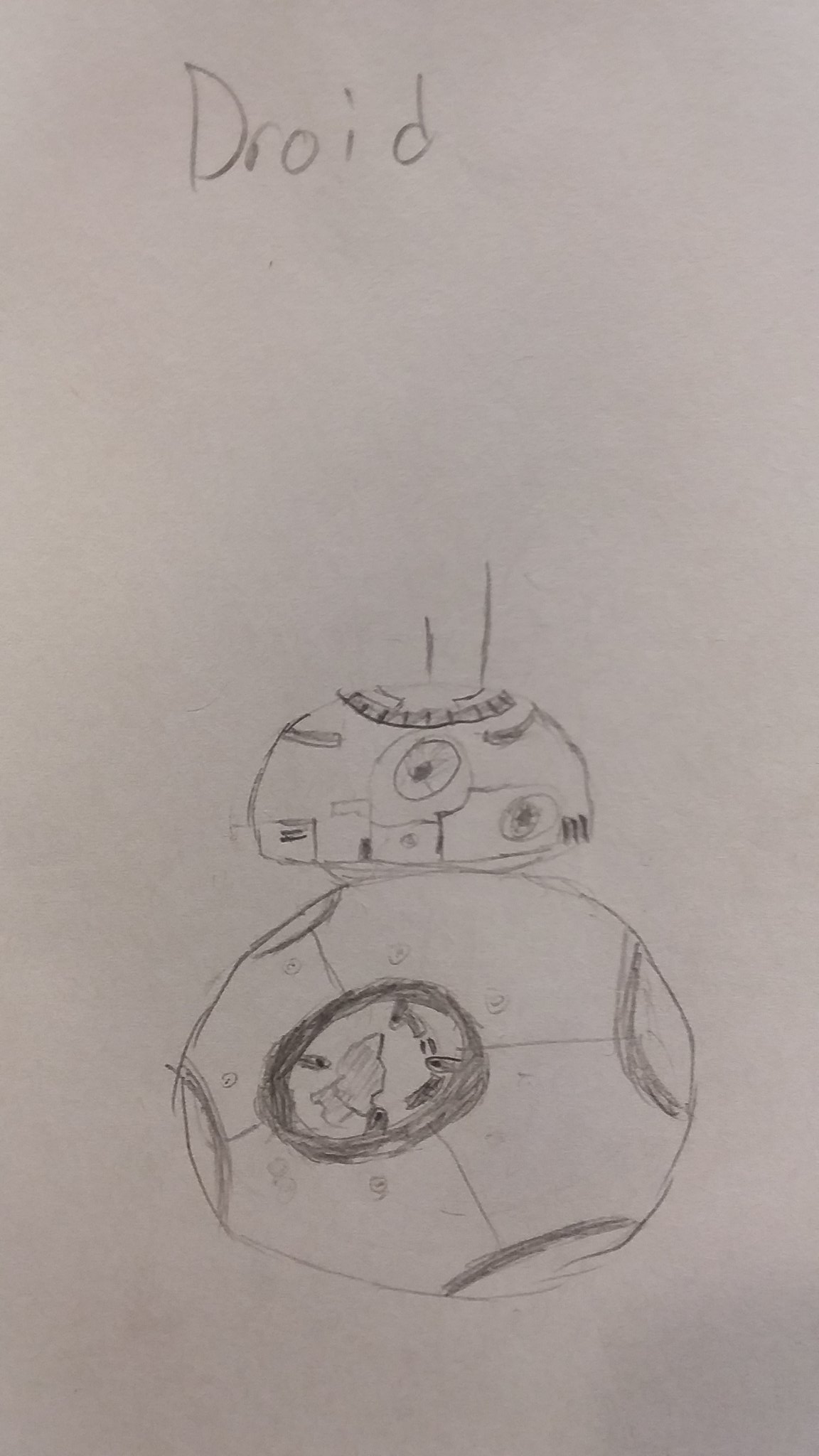A meticulously detailed pencil sketch is drawn on white paper, depicting a stylized droid reminiscent of the iconic red droid from Star Wars. The word "DROID" is inscribed in block letters at the top of the page. The droid's head is illustrated as a large, semi-circular shape with an additional half-circle formed on top. Within this head, two smaller circles are carefully placed. The body is a complete circle, adorned with four half-circles symmetrically arranged around the perimeter. The center of the body features a distinct circle that contains a half-moon shape. Complementing the simplistic, yet precise design, two straight lines of varying lengths protrude from the top of the droid's head, adding an element of dimension to the otherwise 2D sketch.